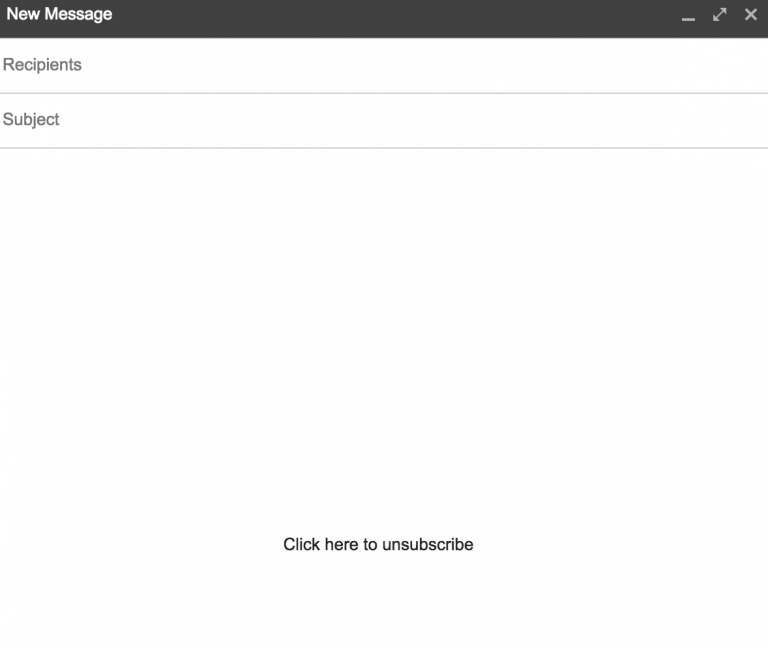Here is a polished and detailed caption for the image described:

"An all-white background is topped by a slim black bar featuring the words 'New Message' in white. To the right side of this bar, there is a white minus sign and a double arrow, slanted and pointing both up and down. On the far right end of the bar, there is a white 'X'. Below 'New Message', the word 'Recipients' appears in a light gray color, followed by a horizontal gray line underneath. The next line displays the word 'Subject'. The middle of the image consists of a large blank space without any lines or text. At the very bottom, in bold black letters, are the words 'Click here to unsubscribe'. The text 'Click here to unsubscribe' is the final element, with no additional text or graphics below it."